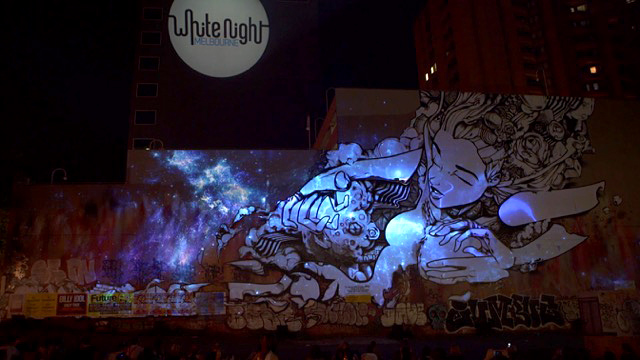The image captures a mural painted on the side of a building during the nighttime, likely in Melbourne, Australia. The artwork is a detailed, anime or sci-fi styled depiction of a woman with closed eyes, featuring an abstract, white-and-black design. The woman appears to have an Asian influence in her facial features and is portrayed with her head leaning back, facing left. Her hair is an intricate mix of what could be flowers or metallic elements, adding an otherworldly aspect to the piece. Her body, particularly her chest, is cupped by two hands, enhancing the surreal, robotic aesthetic of the mural. To the top left, a projection on a nearby building reads "White Night" with the word "Melbourne" prominently displayed below in blue within a white circle, indicating a possible art event. The building hosting the mural is devoid of windows, making the artwork the focal point. Beneath the mural, unreadable yet typical graffiti tags cover the lower part of the wall. The scene includes some figures likely observing the display, emphasizing the public interaction with this urban art installation. The background shows a dark cityscape with varying building heights, adding depth and context to this vibrant street art.